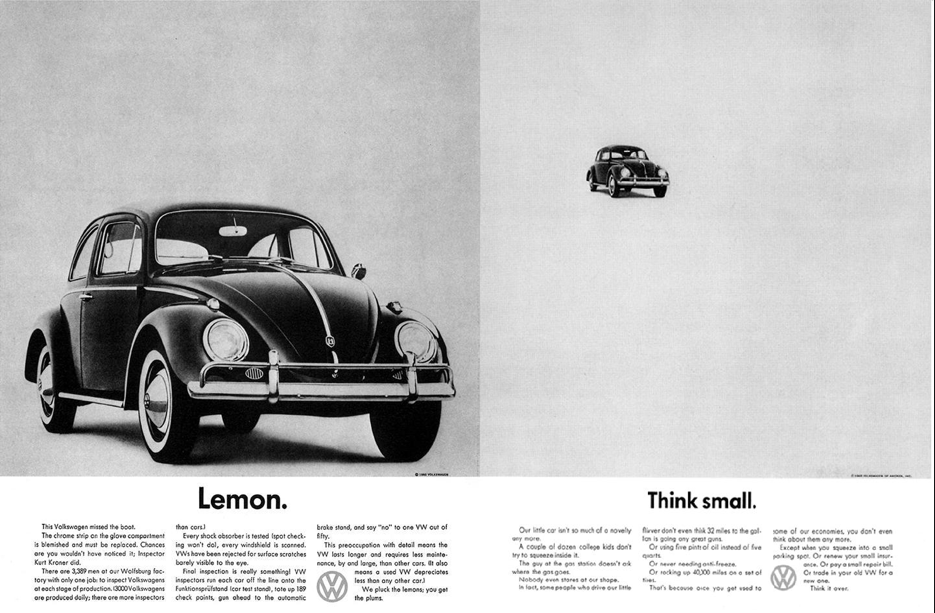The image is a vintage magazine ad for Volkswagen, likely from the 1960s or 70s, split into two pages with distinct details and color contrasts. On the left page, against a darker gray background, there is a black and white picture of a VW Bug. The car, characterized by its round headlights and classic design, is tilted slightly, showing a 45-degree angle. Below the image, bold black text reads "Lemon." This page includes a detailed yet small and somewhat unreadable narrative about Volkswagen's meticulous inspection process, mentioning that every part of the car is thoroughly checked by numerous inspectors to ensure quality. The text emphasizes that flawed vehicles, or "lemons," are removed from production to ensure only the best cars reach customers. Notably, it references an inspector named Kurt Krohner and details about the inspection and testing processes.

On the right page, set against a lighter gray background, the same VW Bug image is displayed, but this time it is smaller and positioned towards the top of the page. Beneath this image, the bold black text reads "Think Small," accompanied by additional fine print that is difficult to decipher. The VW logo is present on the bottom right of each page, adding a final touch to this minimalistic yet impactful advertisement.